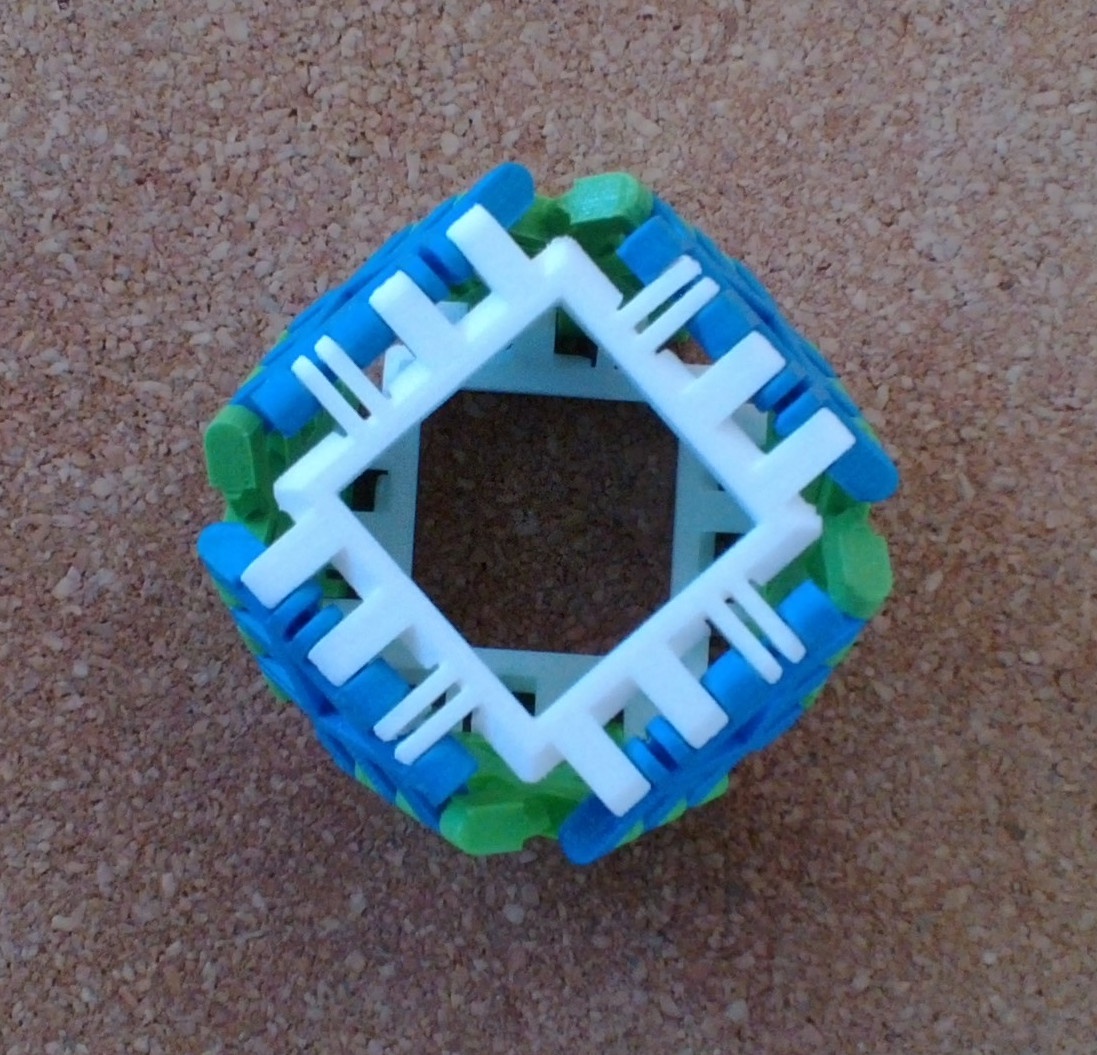The image captures a detailed top-down view of a plastic assembly lying on a richly textured reddish-brown granite-like surface. The granite background features specks of white, grayish-white, and deep red, lending a sense of ruggedness to the scene. At the center of the image lies a complex, white, plastic cube-like structure, potentially an advanced fidget spinner or elaborate 3D puzzle. Each side of this structure has three arms, and four blue components hang off these arms, connected by green connectors. This assembly appears modular, possibly hinged, and may fold or move, suggesting a dynamic toy-like quality. The bottom section of the white structure is visible but presented at a slightly different angle, enhancing the three-dimensional aspect of the assembly. The image quality is slightly blurred, but enough detail is visible to appreciate the intricacy of the design, which includes tabs on the plastic parts allowing them to fit together snugly, akin to a 3D-printed Lego formation.